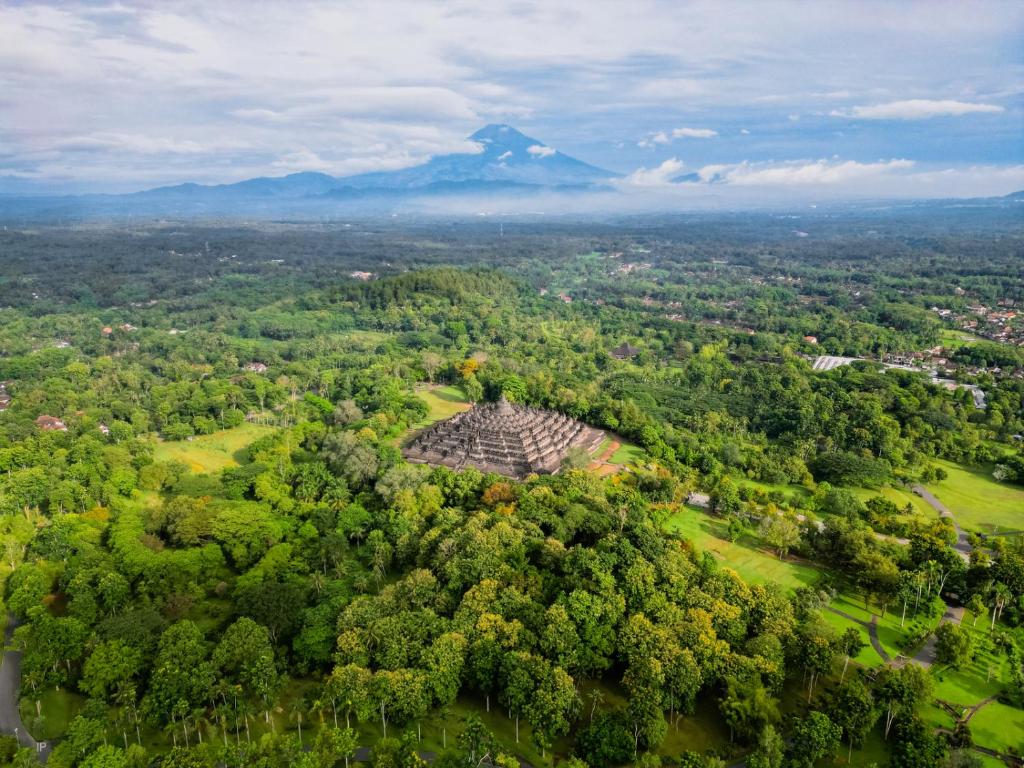An aerial color photo captures an expansive, verdant landscape teeming with green trees of various shades and heights, forming a dense, forest-like environment. The central focal point is a gray, pyramid-like stone structure that resembles a unique temple with tiered steps ascending its height. Towards the distance, the canopy gives way to browner, more barren areas, likely due to the elevation of an approaching mountain range. These mountains, blue-tinged from the sky's reflection, decrease in height from the center to the sides of the image. The sky overhead is a light blue adorned with scattered white clouds, suggesting a sunny day. Sunlight glistens subtly on the landscape, particularly noticeable in the bottom right and central regions. In the far right background, hints of a human settlement with scattered houses punctuate the sea of greenery.